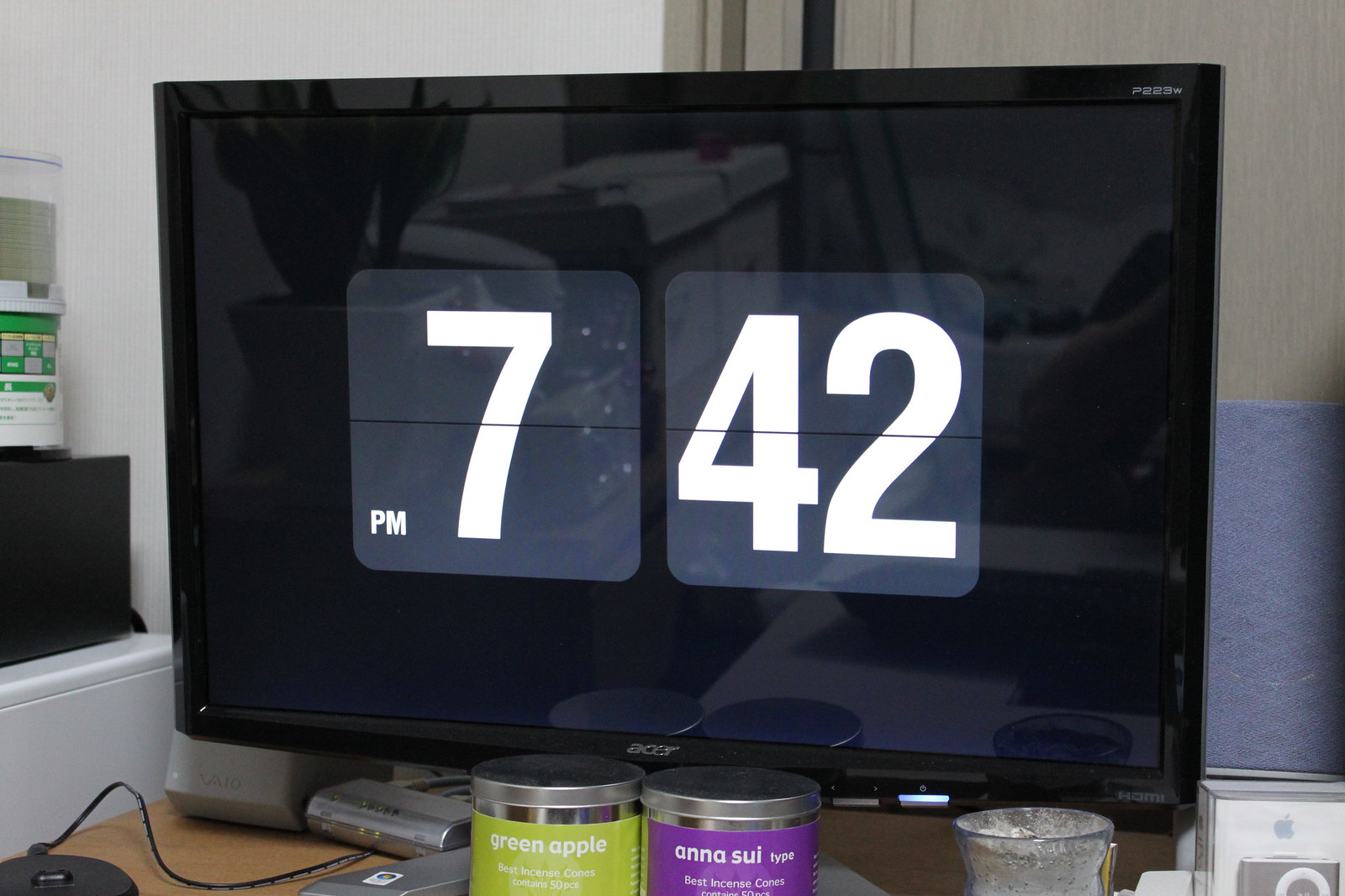This image features a large Acer computer monitor with a sleek black frame. The screen prominently displays a digital clock in the center showing the time 7:42 p.m., with white numbers "7" and "42" inside translucent squares with rounded corners. The monitor's power button is glowing, and there are buttons along the bottom edge. The Acer logo is centered at the bottom of the frame, and the model identifier "P223W" is visible at the top right, while "HDMI" is marked at the bottom right. The monitor is placed on a desk, which also holds two jars of incense—one with a green label for Green Apple and another with a purple label for Anise Soup, both capped with silver lids. Additionally, there is an Apple charging dock on the bottom right, speakers, and various charging equipment behind the monitor. The black background of the screen shows a reflection of some plants in a messy room.